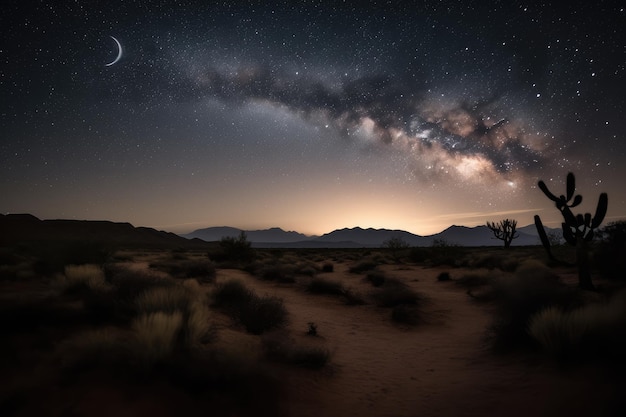This image captures a serene, nighttime desert landscape with a wealth of intricate details. The foreground showcases a sandy terrain dotted with dark green, round shrubs and the silhouetted forms of cacti and Joshua trees. The sand is a muted brown, reflecting the arid environment. In the distance, a small mountain range stretches along the horizon. Above this range, the sun is setting, casting a whitish-gold hue that gradually gives way to a dark, starry sky. The sky itself is a deep black and blue, punctuated by the faint glow of stars and the Milky Way Galaxy with its cloudy, nebulous appearance. Positioned in the top left corner is a slender crescent moon, adding a final touch to this tranquil, post-dusk scene. Little wisps of cloud drift across the center of the sky, enhancing the overall ethereal quality of the night.